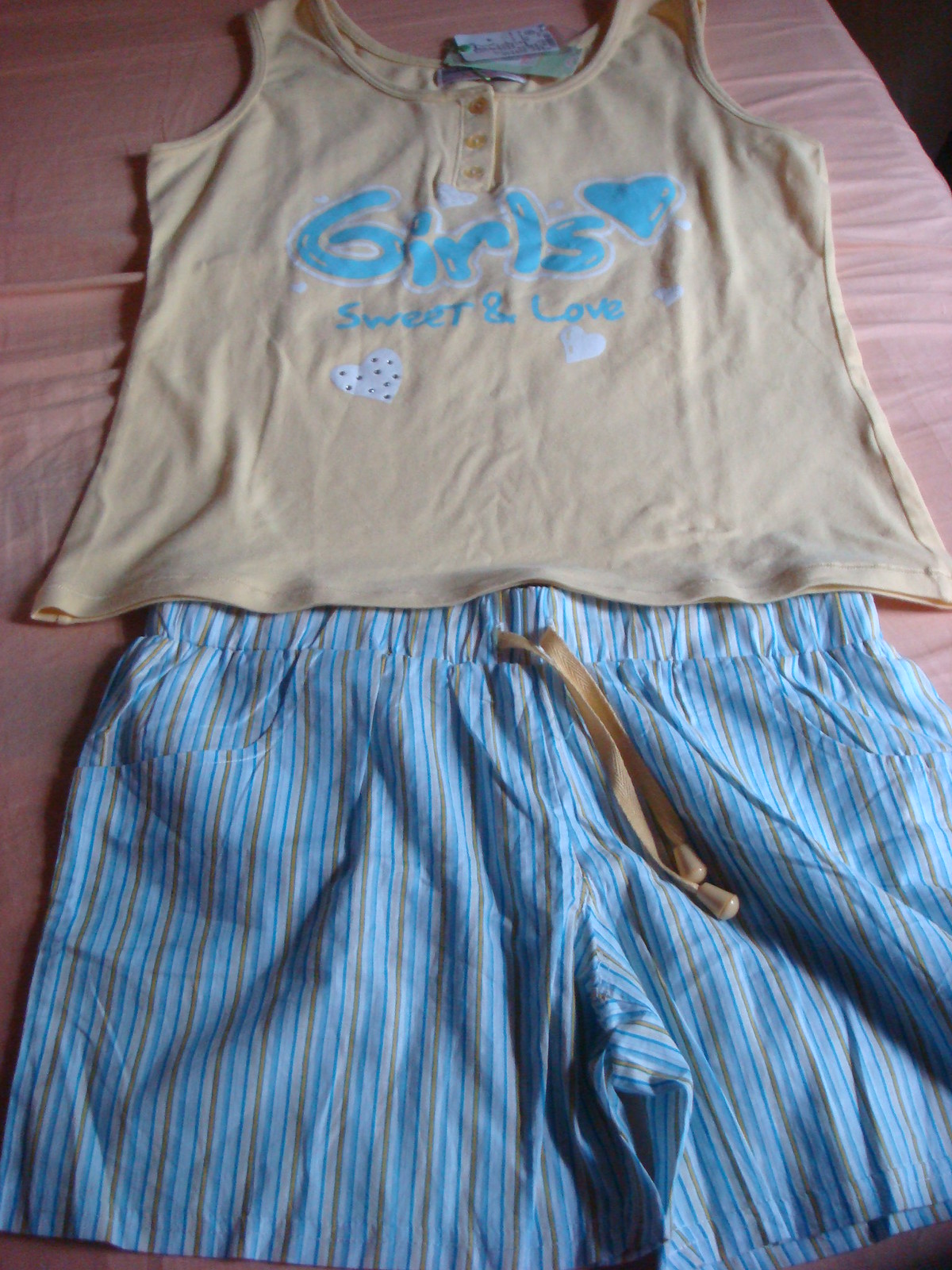In this detailed indoor image, taken in what appears to be someone's bedroom, we see a bed covered with a light pink bedsheet, illuminated enough to contrast with the darker background. The central focus of the photograph is a neatly arranged outfit laid flat on the bed. At the top of the image is a pale yellow (or tan) tank top, designed for a child, with three buttons on the neckline and a visible tag, indicating it is brand new. The tank top features blue lettering that says "girls" accompanied by a blue heart, with additional words "sweet" and "love" written below, surrounded by small white hearts. Below the tank top are striped shorts with a drawstring. The shorts have a light blue background with pinstripes in white and very light brown, and cream-colored drawstrings with caps at the ends. The shorts and tank top ensemble forms a complete outfit, suggesting it might be intended for a young girl. The colors visible in the image include black, pink, yellow, light blue, white, brown, and tan.